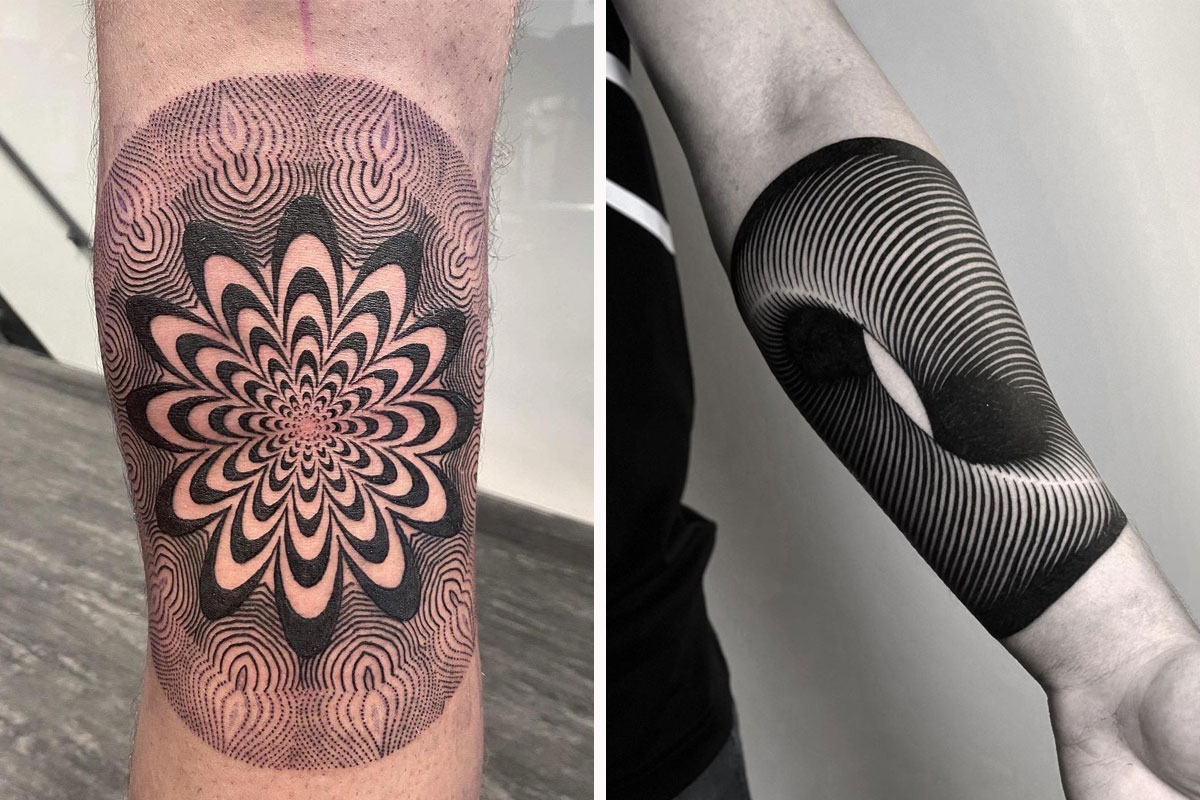The image is a collage of two photographs showcasing intricate tattoo designs on limbs. The left photograph, in color, features a light-skinned individual's leg, specifically the calf area below the knee, adorned with a mesmerizing black tattoo. This tattoo resembles a radiating flower or kaleidoscope pattern, creating a hypnotic effect with its intricate lines and circular arrangement. The background includes a gray wall and a wooden surface. In contrast, the right photograph is black and white, depicting a Caucasian person's extended forearm. This limb is covered in a detailed tattoo that gives the illusion of a 3D spiral, creating the effect of a hole at the center. The arm is shown against a gray wall, and the individual is wearing monochromatic clothing. Both tattoos, though different in design, share a captivating and illusionary quality, emphasizing artistic complexity.